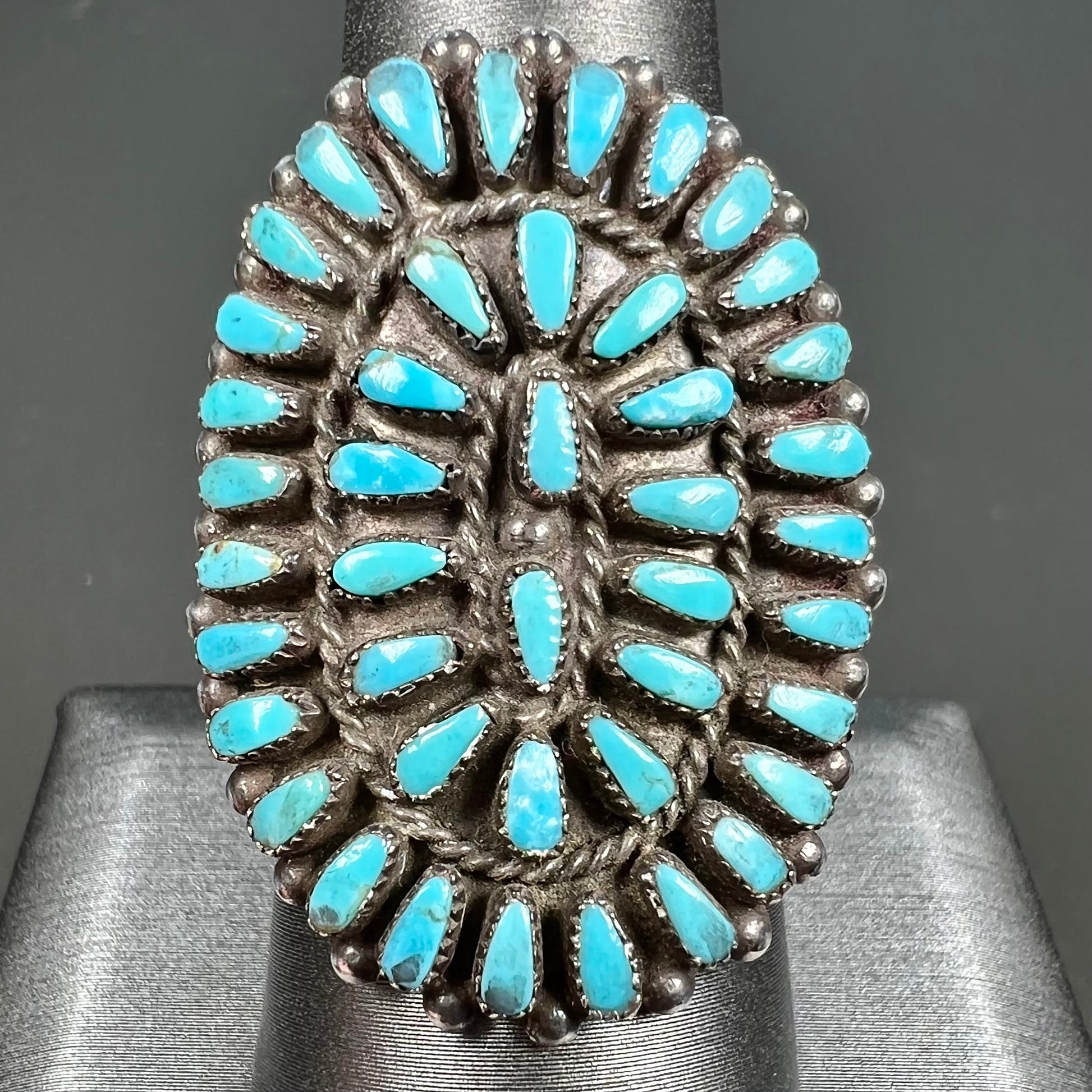This close-up photograph showcases a meticulously crafted piece of jewelry, likely inspired by Southwest Indigenous design, featuring an intricate arrangement of turquoise gemstones. The jewelry forms an oval shape with two concentric rings of small, teardrop-shaped turquoise stones. The outer ring comprises approximately 27 to 28 turquoise stones, each with the point of the teardrop facing inward, creating a striking visual effect. Inside, a slightly smaller inner ring mirrors this pattern with about 16 to 17 teardrop turquoise stones. Nestled between these two oval layers are two additional turquoise pieces, placed side-by-side vertically with their rounded edges facing each other. The entire arrangement is set in a dark, antiqued silver or metallic base, resembling traditional Navajo techniques. This photograph may be part of a museum archive, potentially demonstrating the intricate artistry and cultural significance of such jewelry. The jewelry piece, whether a ring, brooch, or part of a bolo tie, is photographed on a gray metallic stand, highlighting its exquisite detail and craftsmanship.